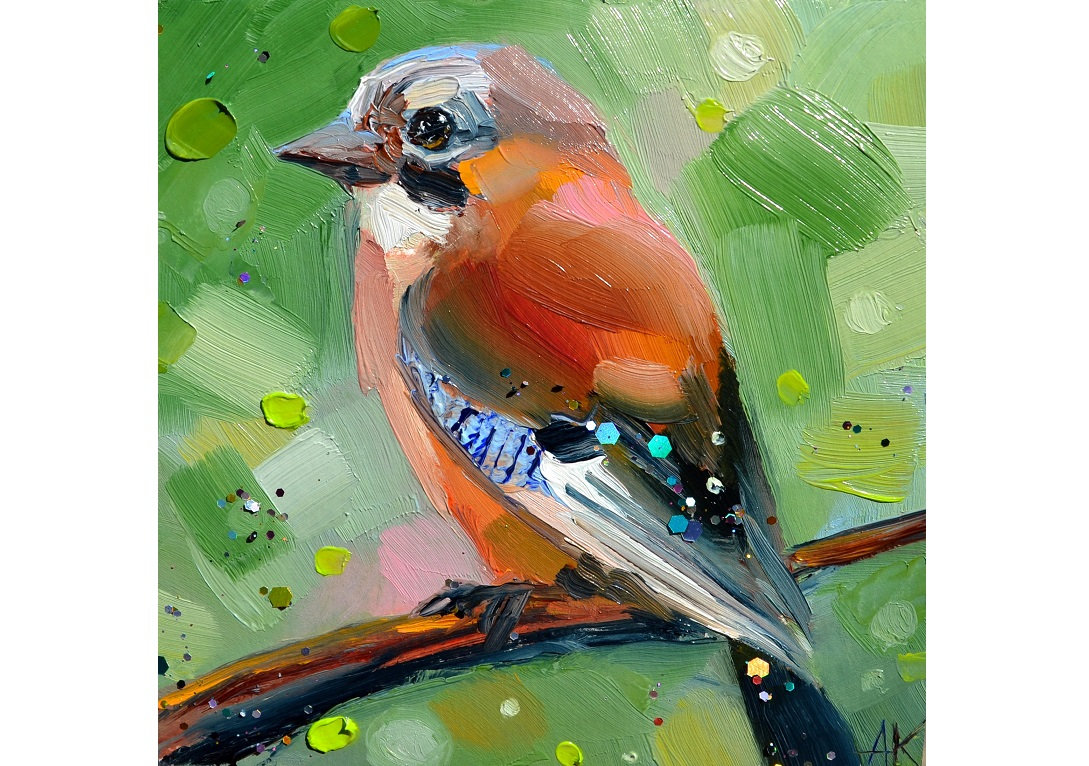This painting, likely executed in oil with large, thick brush strokes, depicts a vibrant bird predominantly colored in shades of red and orange. Its head and wing tips feature various hues including blue, white, gray, and black. The bird is perched on a brown limb, which appears to be a tree branch or stem. The background is rendered with dynamic, glossy green strokes interspersed with touches of a pinkish hue, suggesting a rich, textured environment possibly evoking a sense of rain. Details on the bird's back and tail wings include multicolored hexagonal shapes in teal, light blue, and yellow. The composition is signed with the artist's initials, "AK," in the bottom right corner. The bird is oriented facing left, and the overall brushwork highlights a textured, layered technique across the entire canvas.